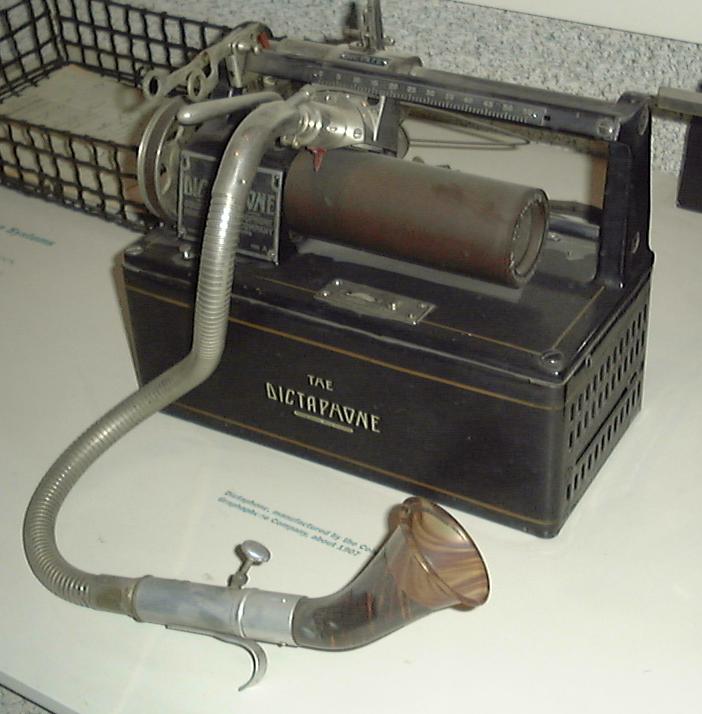This detailed image showcases a vintage dictaphone, a notable early recording device. The contraption resembles a toolbox with a large brown metal body adorned with “The Dictaphone” inscribed in an angular, white font. Prominently, there is a movable needle apparatus, bound to a part that can traverse a central spinning cylinder, akin to a rotating drum. Extending from one end of this needle mechanism is a hose, which culminates in a brown glass mouthpiece. Users would speak into this cup-like mouthpiece, allowing the vibrations and sound waves to be etched onto the rotating cylinder, enabling voice recording and playback. The entire piece exudes an archaic charm, covered in dust and resting on a white table, evoking images of an early speakerphone prototype.